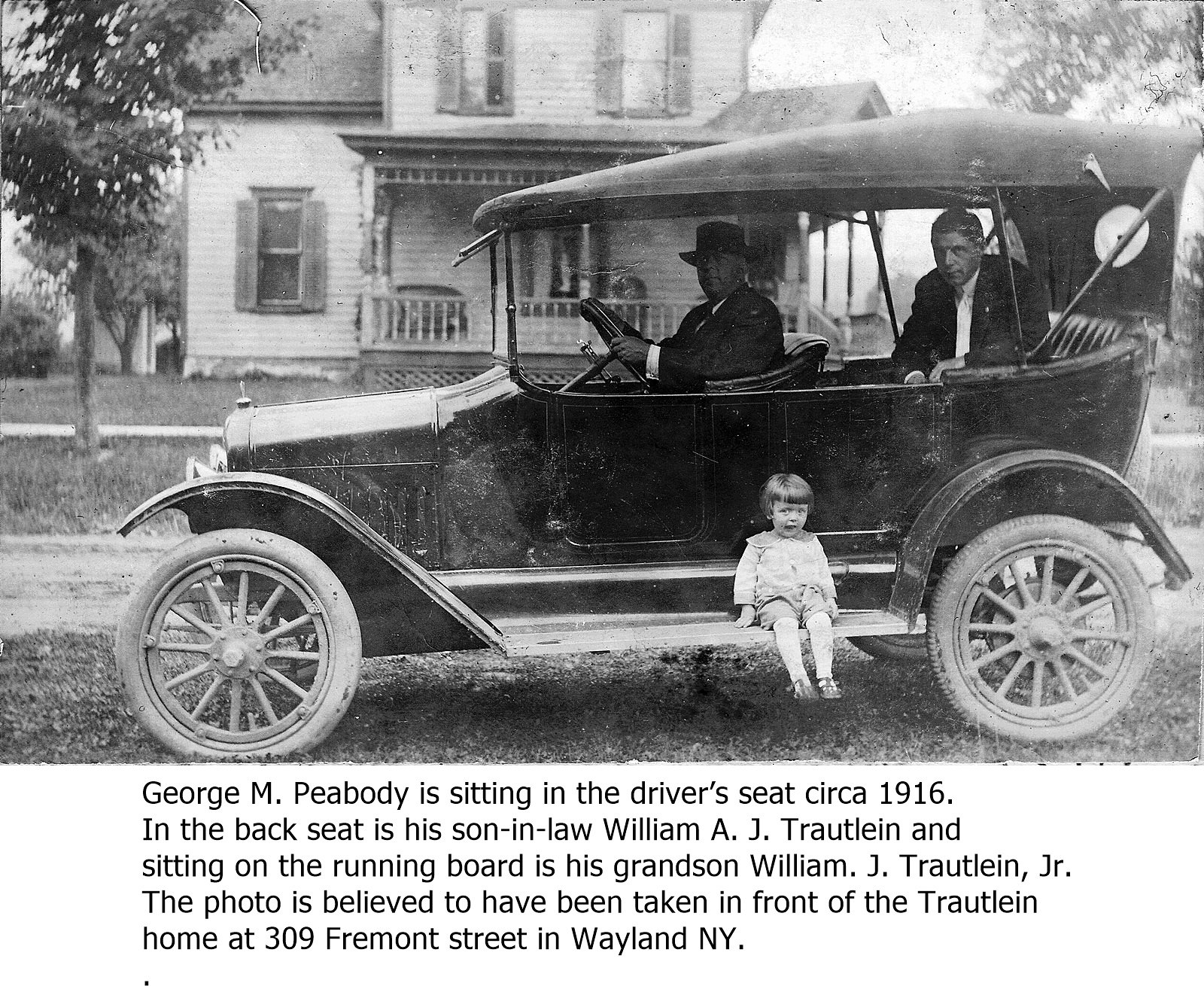This black and white photograph, dating back to circa 1916, features an old Model T-type car facing left. The car, characterized by its black color, cloth top, and skinny tires, is parked on what appears to be a street outside a Victorian-style house, likely at 309 Fremont Street in Wayland, New York. George M. Peabody, dressed in a suit and black top hat, is seated in the driver's seat. In the back seat, his son-in-law, William A.J. Troutlian, also wearing a suit, is slightly turned towards the camera. Sitting on the sidestep (also referred to as the running board) of the vehicle is Peabody's grandson, William J. Troutlian Jr., a small girl dressed in light clothes and stockings. Additional background details include a front porch, a tree, and grass on the sidewalk, enhancing the nostalgic and historic ambiance of the image. Beneath this rectangular photograph are five lines of black print that provide the names and relationships of the people in the car, as well as the believed location of the photo.